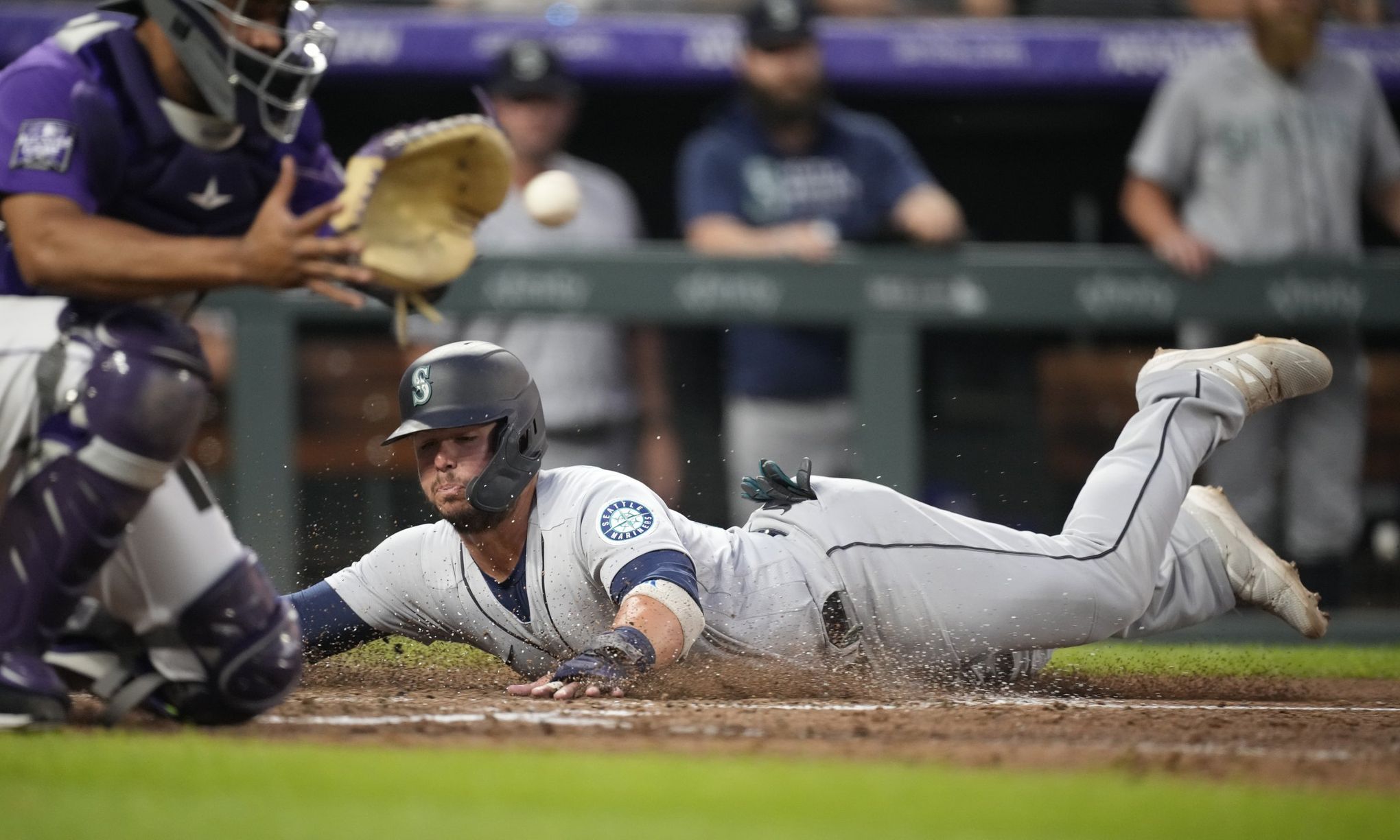This action-packed photograph captures the intense moment of a baseball player sliding into home plate. The player, likely from the Seattle Mariners, is fully extended on the ground, kicking up a cloud of dirt as he slide across the base path. He wears a black helmet with an 'S' on it, and his white uniform features blue highlights and stripes running down the sides of his pants. Both his legs are airborne as he stretches out to touch home plate, his face a picture of determination. 

Positioned to the right is the catcher, clad in purple protective gear, making a desperate attempt to catch the incoming ball. He is squatting on one knee, his mitt outstretched as the baseball hovers mere inches away, indicating it's a very close play. In the blurred background, the Seattle Mariners' dugout can be seen along with several spectators, emphasizing the focus on this critical moment. The player's dramatic slide and the catcher's reaction create a moment of palpable tension, suggesting the player might just have made it home safe.